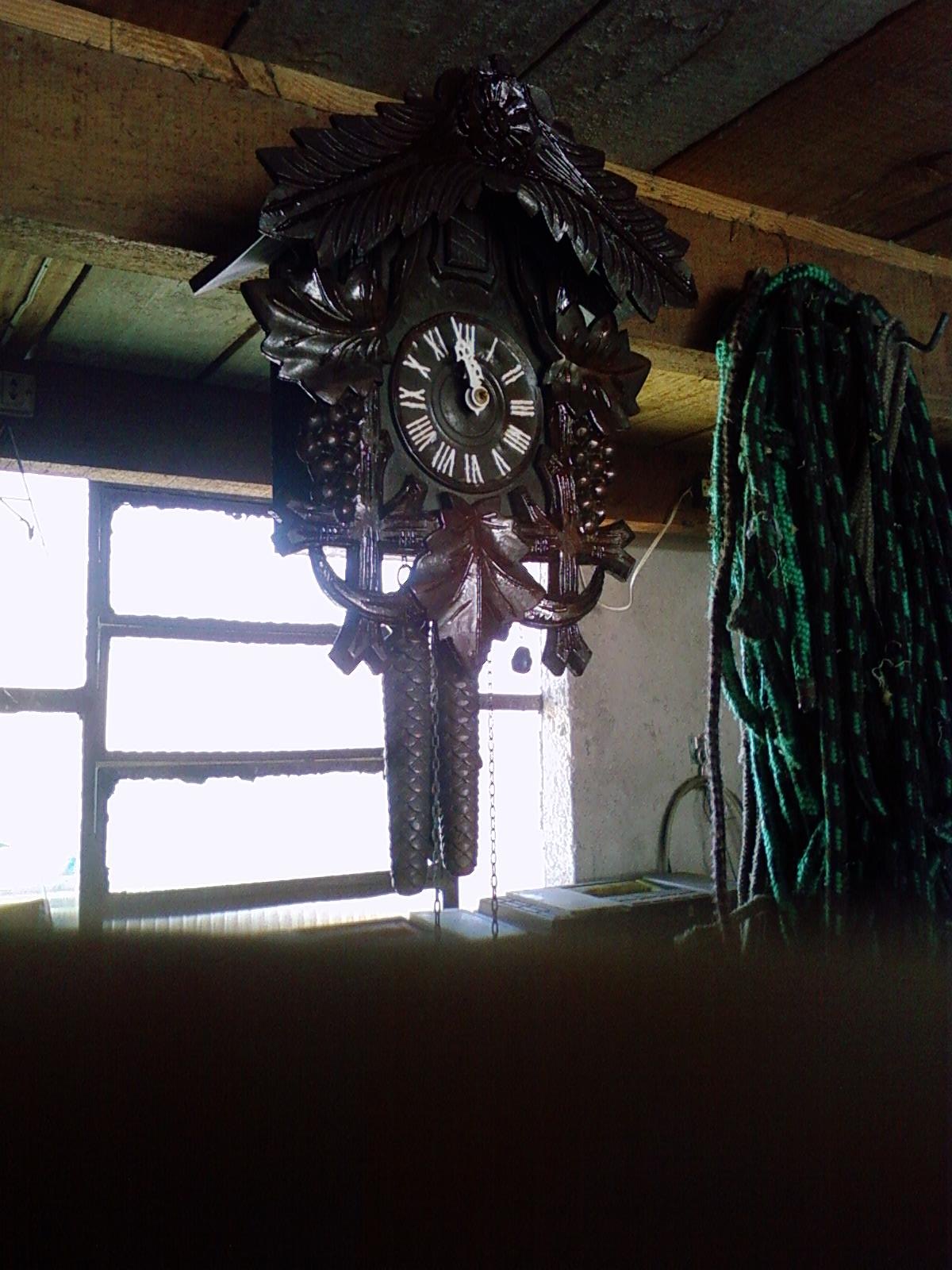In this photograph set in what appears to be a dimly lit workshop or barn, an intricately carved cuckoo clock becomes the focal point amidst a cluttered background. The clock, crafted from dark wood with a rich burgundy or deep purple hue, displays finely detailed engravings. Prominent among these carvings are floral and leaf motifs, as well as figures resembling walnuts or berries. A pair of pine cone-shaped weights dangles below, used for adjusting the time.

The clock face itself is notable for its black background, with stark white Roman numerals and hands that are close to the 12 o'clock position. Above the clock face, a small black window or door likely serves as the entrance for the cuckoo bird. To the right of the clock, numerous green and black striped ropes hang in bundles from a ceiling hook.

The setting is characterized by a mix of wood and possibly metal elements, contributing to an overall rustic aesthetic. A garage door is slightly visible in the top left corner, while an old, paint-chipped window at the back of the room casts natural light into the otherwise dark interior. This light, however, is diffused, possibly indicating an overcast or extremely bright sky outside. Below the window, a small, light gray table stands against the wall, adding to the scene's detailed composition.